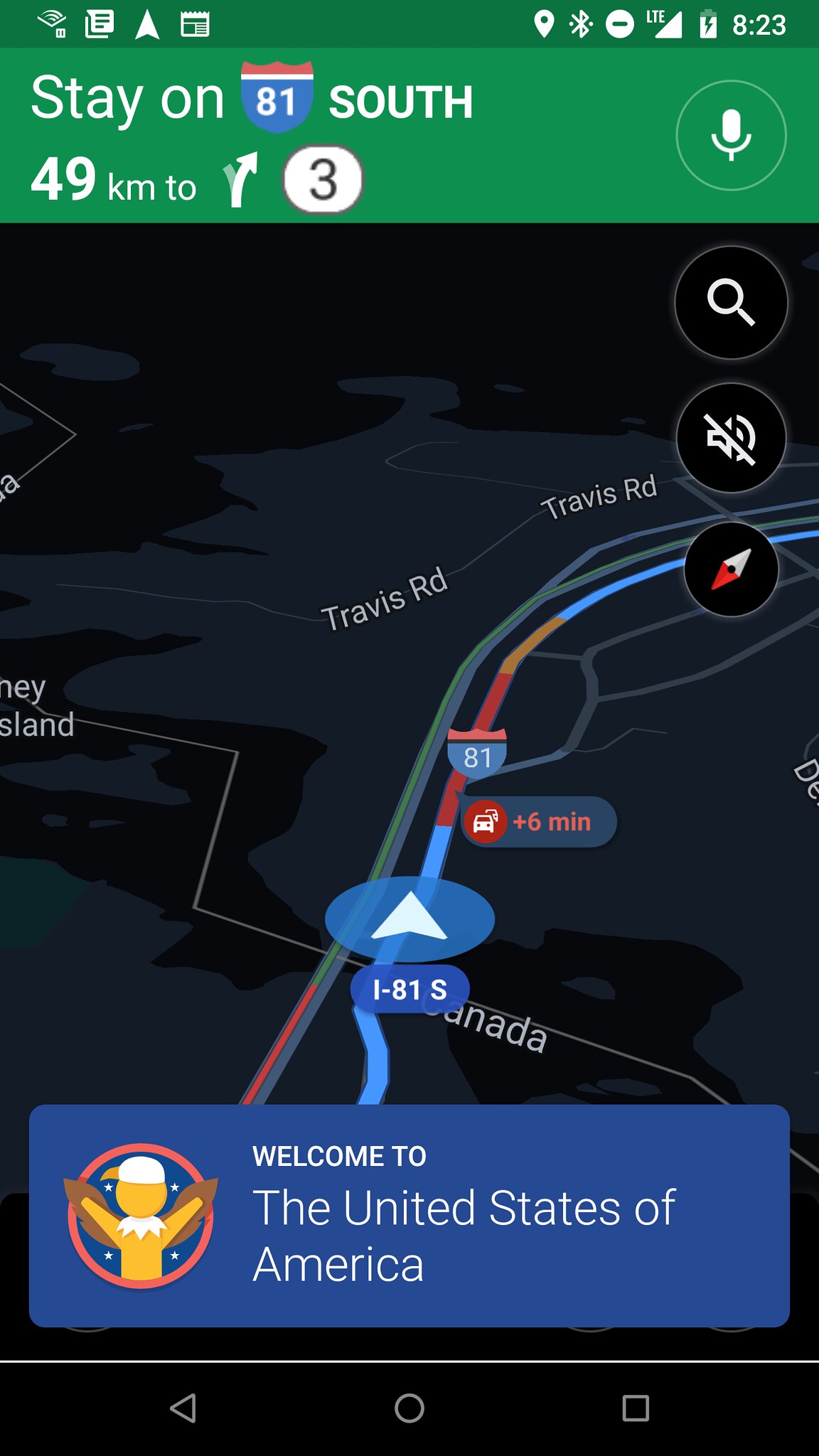The image is a detailed, colorful screenshot from a smartphone, depicting a GPS navigation app, likely Google Maps. The aspect ratio of the image is roughly twice to two and a half times as tall as it is wide. At the top of the screen, standard phone elements such as time, signal strength, and battery level are visible. Below this, a prominent green bar spans horizontally, occupying about 20% of the screen, and displays the instruction "Stay on 81 South." It also includes the route icon with "49 kilometers to Route 3" and an arrow indicating a right turn ahead. 

Beneath the navigation instruction, the map shows the user's current route, where they are entering a congested area marked by red and orange before returning to blue, indicating smoother traffic. Additional circular icons for functions like a microphone, search, and no noise are present. At the bottom, white lettering on a blue background reads "Welcome to the United States of America," indicating the user just crossed the Canadian border into the US. The time displayed on the phone is 8:23 AM, with all elements suggesting good signal strength. Additionally, there's a circle icon depicting a person with raised hands, signaling a congratulatory or welcoming gesture.